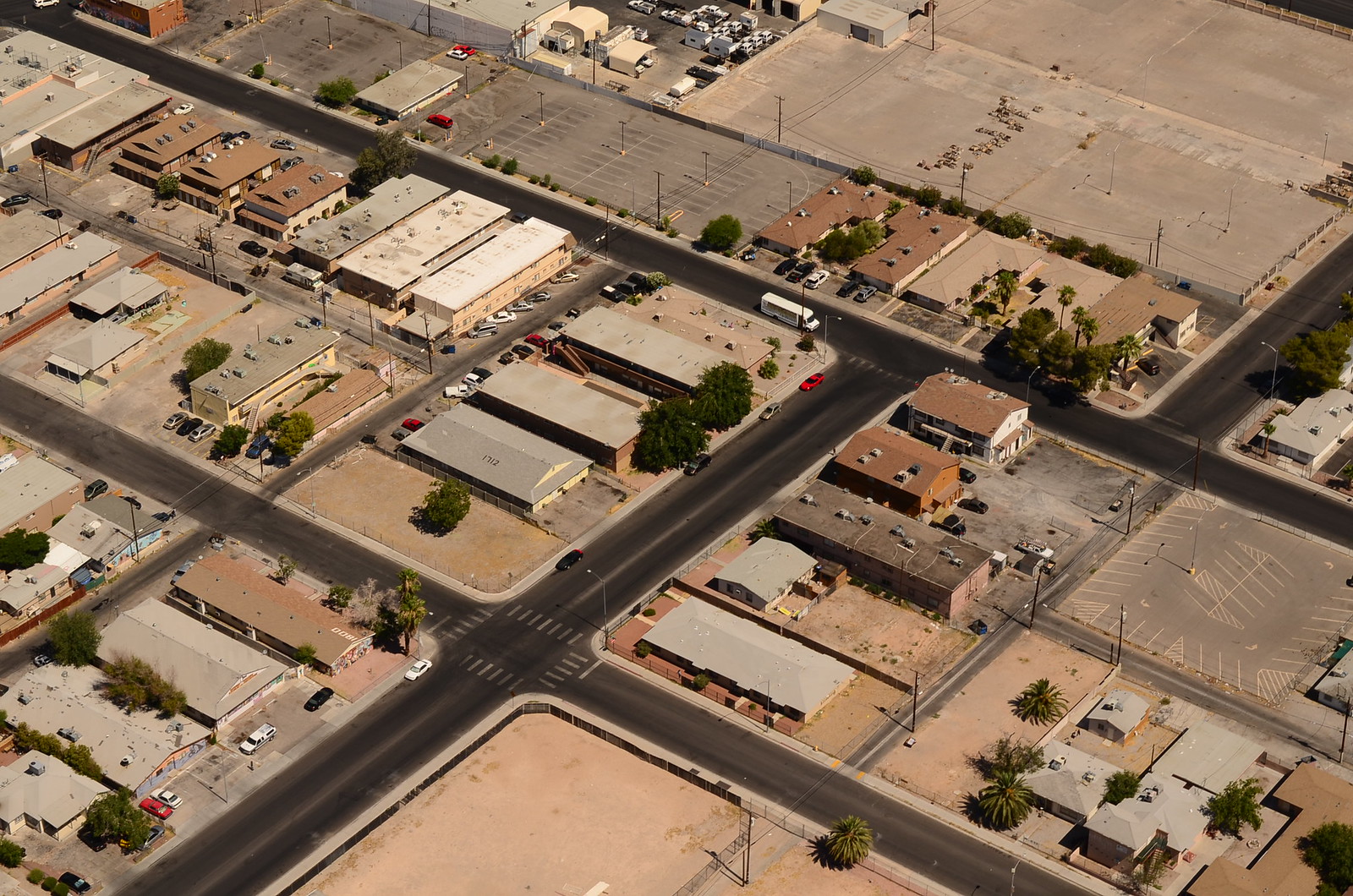A detailed aerial view reveals a semi-industrial area characterized by numerous parking lots and a variety of buildings, primarily businesses and warehouses. The upper right-hand corner prominently features a large parking lot. The landscape is sparse, with minimal tree coverage—only a few scattered trees are visible. Among the buildings are several that appear to be small office structures, possibly housing doctor's offices or similar establishments. A couple of roads traverse the area; one has a truck in motion, but otherwise, the roads are devoid of moving vehicles and pedestrians. All other vehicles are stationary, parked within the various lots. The buildings, which predominantly have light-colored roofs with a few exceptions in reddish hues, are mostly single-story structures with no skyscrapers or tall buildings in sight. The image contains no street signs or visible people, presenting a serene, unpopulated scene focused solely on the industrial and business establishments.